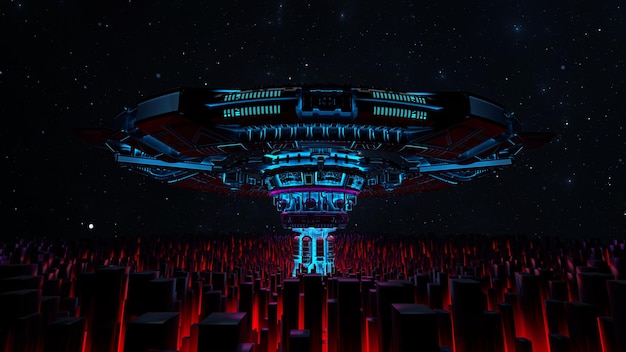A captivating nighttime scene features a massive, disc-shaped spaceship, primarily glowing blue, suspended in a dark, star-filled sky. Its structure includes a cylindrical base and sporadic black and brown details. Centered directly above what appears to be a futuristic city comprised of pyramid-shaped buildings and block-like structures glowing red, the spaceship's blue illumination contrasts dramatically against the varied hues of light purple, dark blue, and white scattered throughout the city below. The cityscape occupies the entire lower half of the image and is bathed in red light, giving the impression of red pedestals or spikes rising from the ground. This visually striking, digital creation emphasizes the alien spacecraft hovering over the city, reinforcing the nocturnal and otherworldly atmosphere captured in the image.